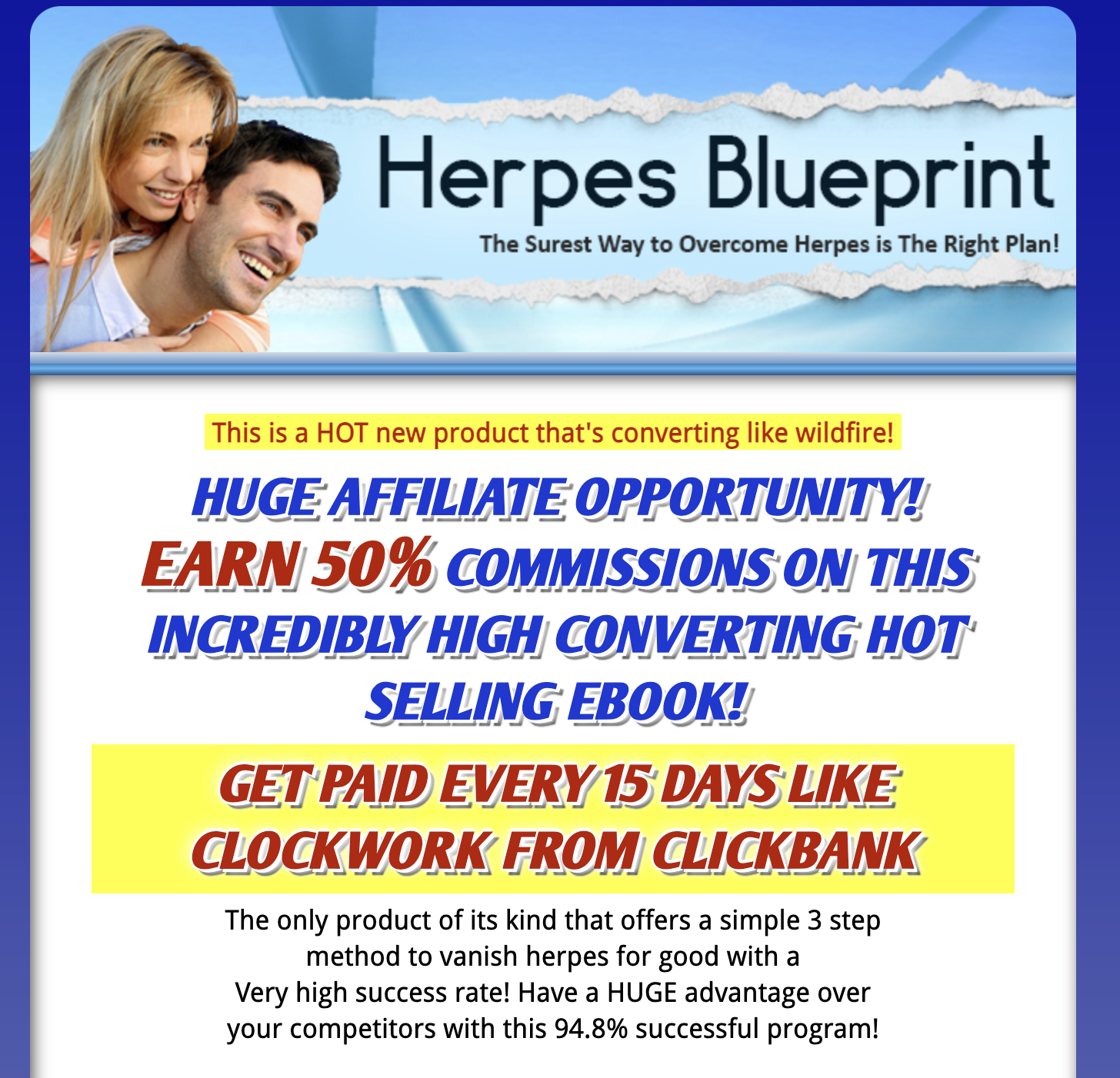**Caption:**

This is a confidential promotional flyer for "Herpes Blueprint," depicting a smiling woman hugging a man from behind. The title "Herpes Blueprint" is prominently displayed in black, with white smoke trails above and below it, and accented with blue elements throughout the flyer. Below the title, the text reads: "The surest way to overcome herpes is the right plan." The flyer features vertical blue borders on both sides and additional white smoke effects. 

Highlighted in yellow is an attention-grabbing phrase: "This is a hot new product that's converting like wildfire." In bright red text, it states: "Earn 50% commissions" followed by the note that this is an "incredibly high converting hot selling ebook." It further mentions that affiliates get paid every 15 days through ClickBank, highlighted in yellow.

The flyer emphasizes in black text that this is "the only product offering a simple three-step method to eradicate herpes for good," boasting a remarkable 94.8% success rate. It encourages affiliates to leverage this high success rate for a significant advantage over competitors. All of this promotional content is set against a clean white background.